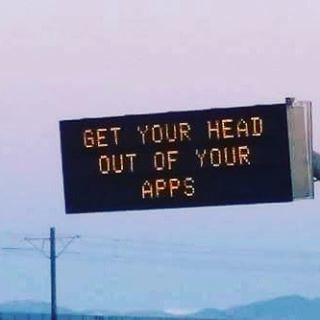The image portrays an electronic sign with a black background and bold, uppercase orange letters illuminated against it. The sign, reminiscent of those typically seen on interstates or highways providing travel information, instead displays a playful yet stern advisory: "GET YOUR HEAD OUT OF YOUR APPS." This message stands starkly visible against a picturesque backdrop of the setting sky.

The sky, captured at dusk or twilight, exhibits a serene and gradual transition of colors. At the top, a delicate pink hue blends seamlessly into a pastel light blue, evoking a tranquil and comforting atmosphere. Below this soft gradient, the sky meets a distant range of blue-gray mountains, which appear hazy, suggesting a peaceful but slightly obscured horizon.

Stretching beneath the electronic sign and in front of the mountains, a series of power lines subtly intersect the scene, adding an industrial element to the otherwise natural landscape. The overall composition is a striking juxtaposition of modern technology and timeless natural beauty, all under the serene cloak of the fading light.